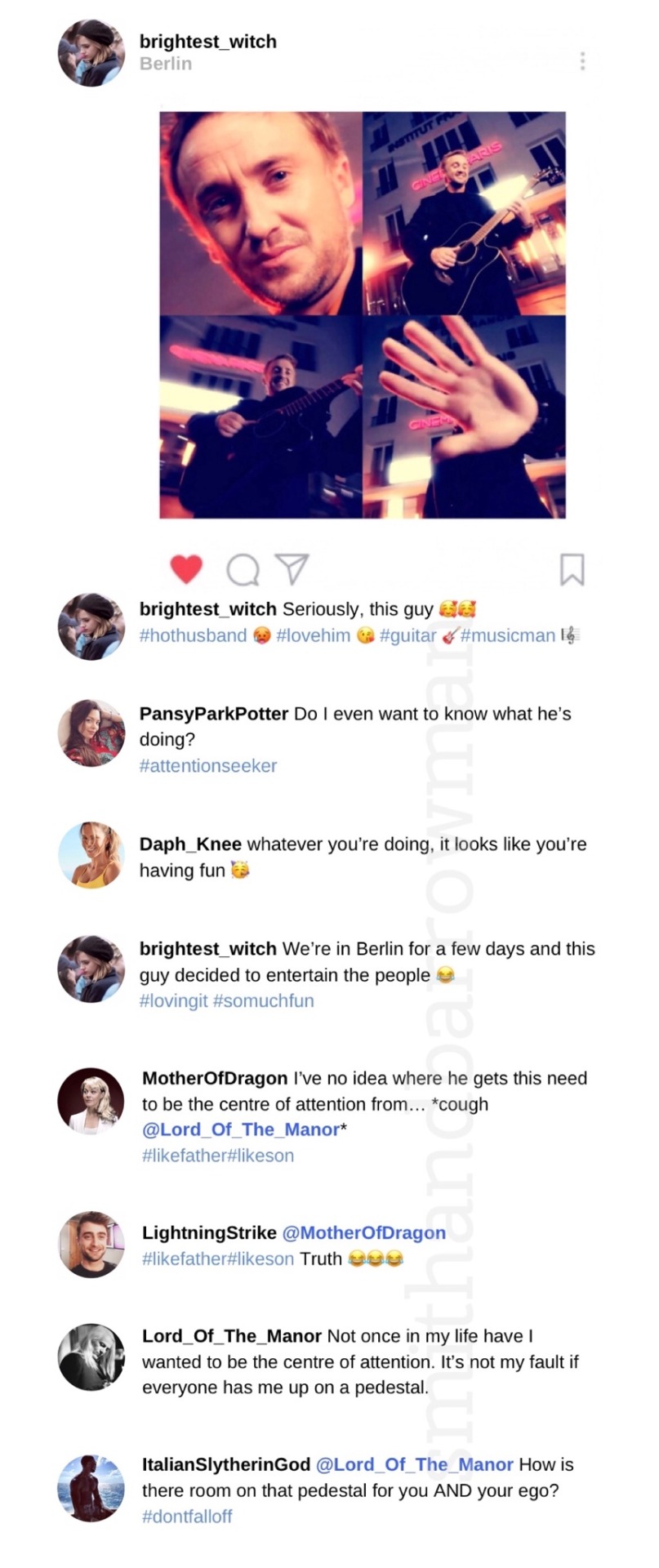**Detailed Descriptive Caption:**

This image is a screenshot of a Twitter conversation featuring several participants engaged in an exchange of messages. The background of the Twitter interface is white. In the top left corner, there's a circular profile picture of a girl dressed in a black ball gown and a black jacket. Adjacent to her photo, her username is displayed as ‘brightest_witch’ in black text, with ‘Berlin’ written underneath in gray.

Below her profile information is a collage of four images forming a single composite picture. The first image in the top left quadrant shows a close-up of a man with blonde hair and some beard stubble, looking directly at the camera. The top right image reveals the same man standing outside, in front of a white building while playing a black guitar. The bottom left image is a closer shot of him playing the guitar in front of the building. The bottom right image shows the man reaching towards the camera with his hand, partially covering the lens, with the white building still visible in the background.

Underneath this collage, several icons appear from left to right: a red heart (like), a speech bubble (comment), a share icon (retweet), and a bookmark icon.

Following this is a threaded conversation. The same profile picture of the girl in a black gown reappears with her response, which includes four hashtags and some emojis. Another user, a woman with long hair and wearing a red shirt, named Pansy Parker Potter, contributes a single line followed by a hashtag. Next, a blonde-haired girl in a yellow shirt, username 'deaf_knee,' responds with two lines. The original poster, ‘brightest_witch,’ replies again with two lines and two hashtags. 

Subsequent replies include a girl with a black background, wearing a white shirt and with blonde hair, named 'mother_of_dragon,' who responds with two lines and tags the user 'lord_of_the_manner,' adding a hashtag. The conversation continues with 'lightning_strike,' a dark-haired man who mentions 'mother_of_dragon' and includes another hashtag. Following this, another user with blonde hair and the same username 'lord_of_the_manner' writes back with three lines. Lastly, there's a man sitting outside, with an Italian vibe, using the username 'italian_slithering_god,' who contributes two lines to the discussion.

This detailed interplay of images and comments showcases a vibrant and interactive conversation among friends and followers on Twitter.